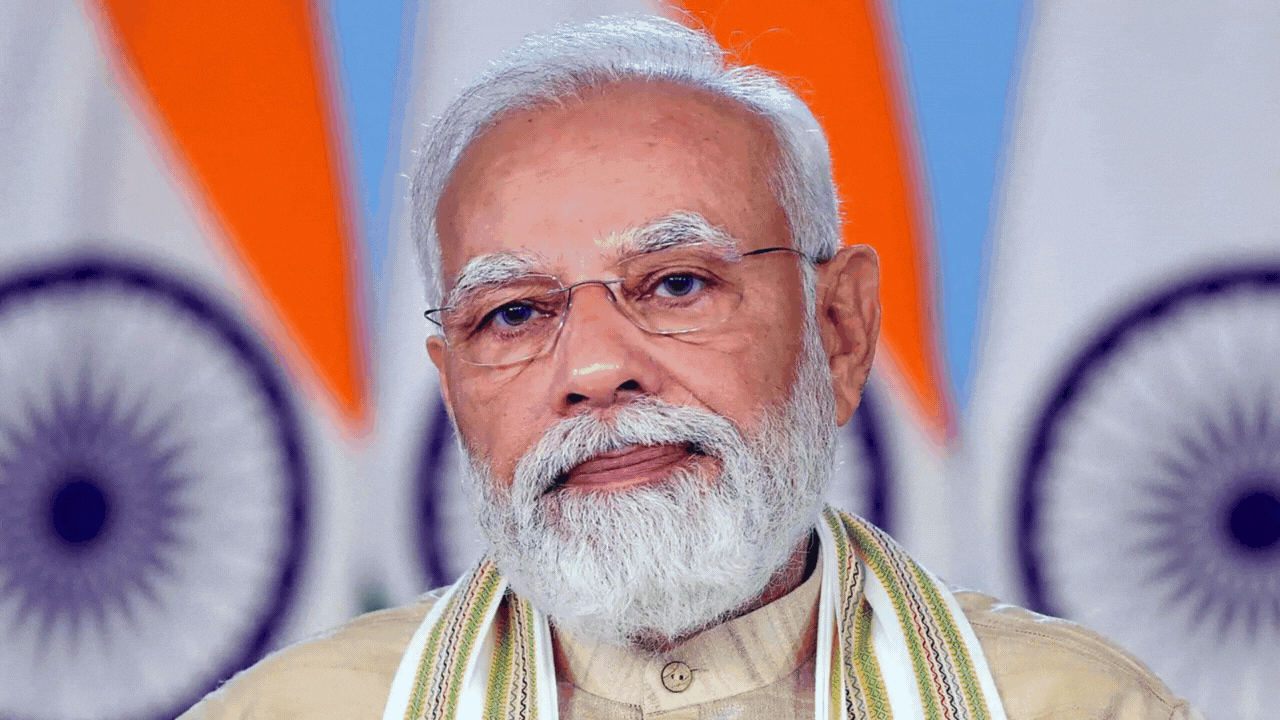This color photograph alternates between two distinct images. The first image features an older Indian man with white hair, a mustache, and a beard. He wears glasses and is dressed in a beige or tan shirt with a white scarf adorned with green and white trim. Behind him is a backdrop featuring a mix of floral designs in purple on a white background, along with vibrant shades of orange, blue, and white. The second image captures a dramatic protest scene. A man, possibly Arab, with a long white beard and a headscarf, stands atop a car, holding a Palestinian flag amidst swirling smoke or tear gas. The protest site is chaotic, with barbed wire, people holding what appear to be video cameras or smoke machines, and a partially visible Yokohama sign in the background. The atmosphere is tense, filled with the smoke that makes it difficult to discern all details clearly. The two contrasting images switch back and forth, highlighting the stark disparity between the serene backdrop of the first and the tumultuous protest of the second.